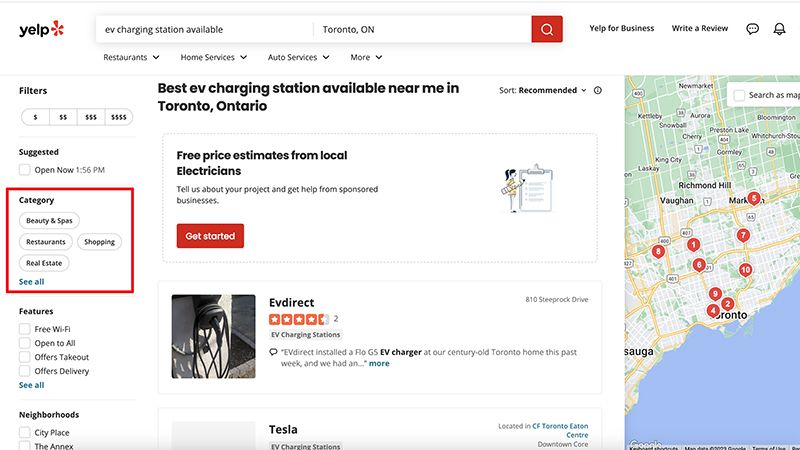This detailed caption describes a screenshot from the Yelp website, providing an extensive overview of its layout and features:

"The screenshot shows the Yelp website interface. The top left corner features the distinctive Yelp logo, adjacent to a search bar with 'EV charging station available' typed in it. Next to the search bar, 'Toronto, Ontario' is specified as the location, followed by a prominent red search icon. Below this, a navigation menu offers clickable options such as 'Restaurants,' 'Home Services,' 'Auto Services,' and 'More.'

Further down, a heading reads 'Best EV Charging Stations available near me in Toronto, Ontario.' Beneath this, a bold announcement offers 'Free price estimates from local electricians,' with a smaller subtext inviting users to 'Tell us about your project and get help from sponsored businesses.' A red 'Get Started' button is prominently placed next to this section.

The section below lists options for charging electric vehicles, featuring 'EV Direct' with a rating of 4.5 stars from 2 reviews, located at 810 Street Brock Drive, along with a single review snippet. Another option listed is 'Tesla.'

On the left sidebar, users can filter search results based on price categories ranging from one to four dollar signs. Additional filters allow toggling between 'Open Now,' examining different categories—such as 'Beauty & Spa,' 'Restaurant,' 'Shopping,' 'Real Estate'—or selecting features like 'Free Wi-Fi' and specific neighborhoods.

On the right side of the page, an integrated map displays the geographic locations of the listed businesses, enhancing the search experience by providing visual context."